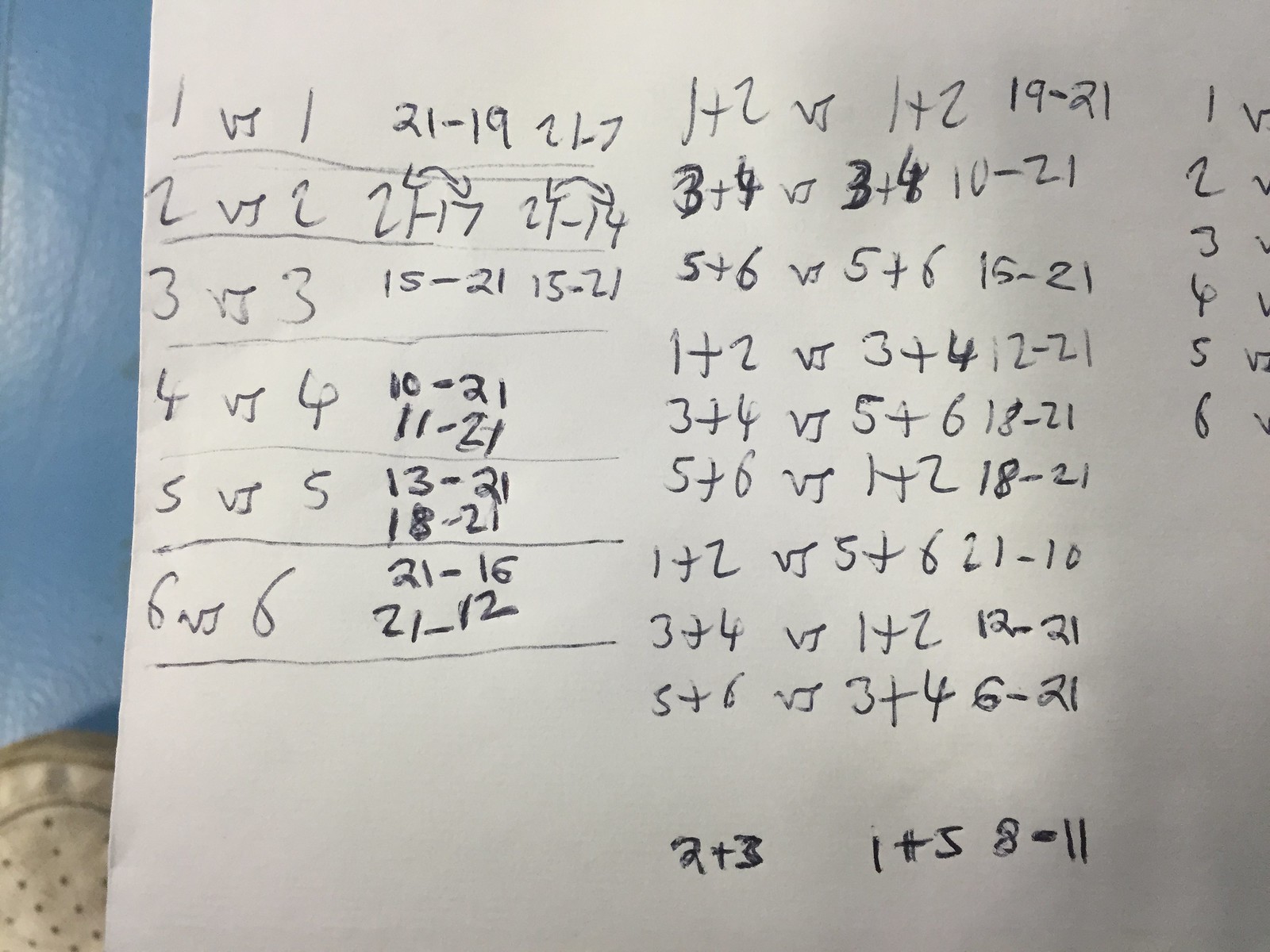A detailed photograph captures a white sheet of paper densely covered in handwritten mathematical equations. The equations, written in black ink, are arranged in three distinct columns. The left column consists of six equations, each meticulously separated by a line to ensure clarity. The central column contains additional mathematical notes, while the right column features another set of equations, partially cropped by the edge of the image.

In the bottom-left corner of the photo, the dirty toe piece of a white trainer is visible, adding an element of casual, everyday context to the image. The background appears to be a textured blue surface—possibly a table or floor—reflecting light in a way that accentuates its raised patterns.

The sheet shows signs of revision, with certain numbers and symbols reinforced to enhance their legibility. This attention to detail underscores the significance of the calculations. The overall composition combines elements of academic focus with personal, lived-in details, offering a glimpse into the process of problem-solving.